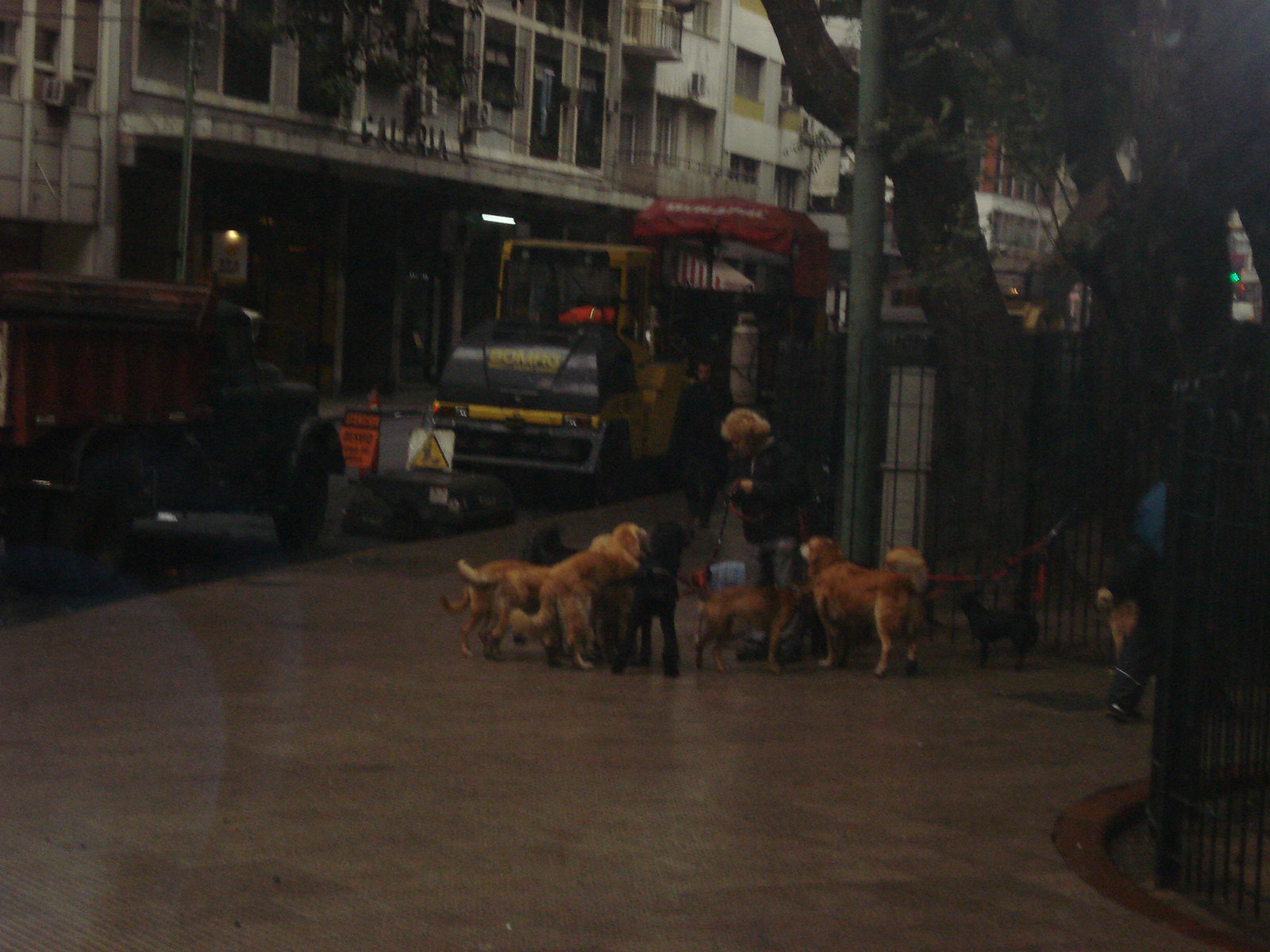In this horizontal, realistic photograph taken outside, the setting appears to be a park entrance, plaza, or a well-maintained sidewalk in a city. The scene is somewhat dim, suggesting it might be a dark, rainy day, which limits the available light and details. On the right side of the image, large trees are bordered by black fencing, and dark brown tiles pave a wide walkway. The focal point is an older woman standing in the center, surrounded by approximately six dogs of varying colors—tan, yellow, and black—likely medium to large in size and furry. Some of the dogs seem to be either golden retrievers or black labs. The woman is holding a couple of leashes, suggesting she might be treating the dogs or preparing for a walk.

Toward the back left of the scene, various vehicles are visible, including what looks like a dump truck and a street sweeper or garbage collection vehicle, evidenced by an arm-like apparatus possibly used for trash pickup. There is also a bus and a construction warning sign indicating a closed road, suggesting ongoing road work. In the background are old, concrete, and stone buildings that appear to be apartments. One significant building has a marquee or overhang with the word "Galleria" prominently displayed in black letters. Another person with multiple dogs on leashes is visible striding in from the right side of the image, hinting at the presence of professional dog walkers in the area.